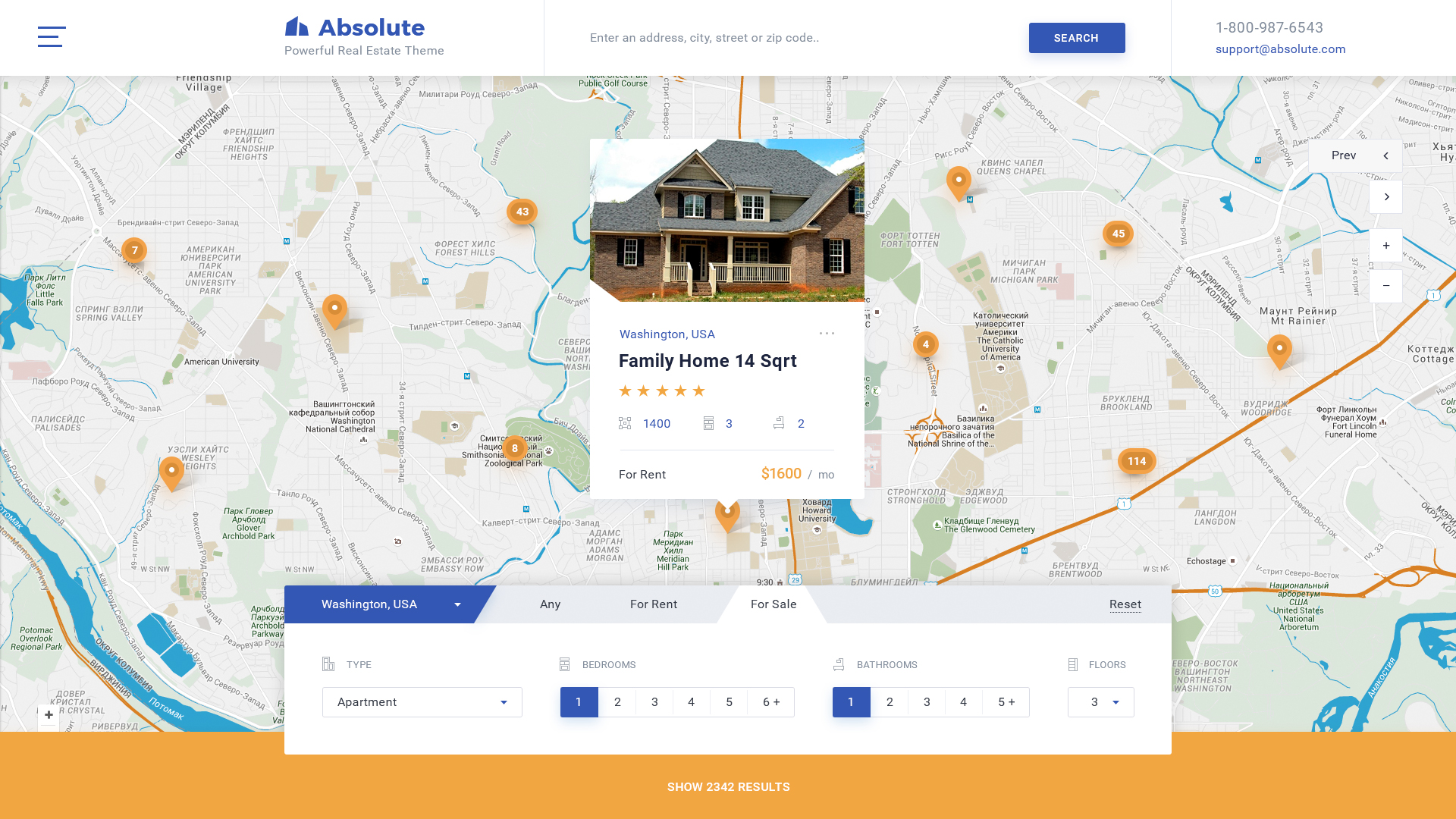This image features a detailed map of a neighborhood with a specific house highlighted, indicating potential interest. The map is overlaid with an interface from Absolute Powerful Real Estate, showcasing a theme promoting real estate options. The top part of the screen reads "Absolute Powerful Real Estate Theme." There's a search bar for entering addresses, cities, streets, or postal codes, accompanied by contact information: phone number 1-800-987-6543 and email support@absolute.com. The map indicates the location in Washington, USA, and highlights a family home with critical details: 14 square feet, five-star rating, and a fast rent option at $1,600 per month. Users can toggle dropdown menus to filter results by rental or sale status, property type (apartments, houses), number of bedrooms (defaulted to one), bathrooms (defaulted to one), and floors (currently set to three).